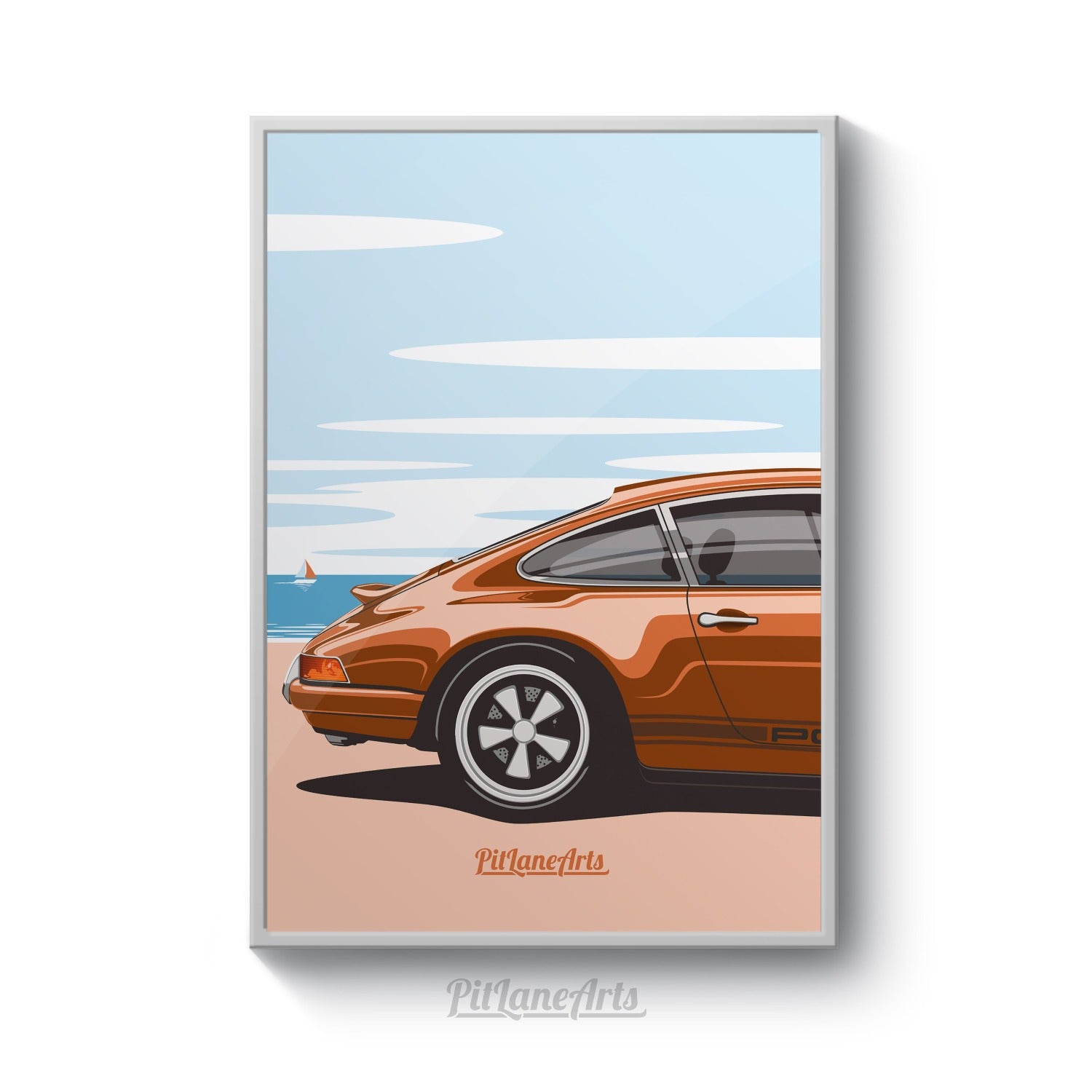This image is a vertical photograph of a modern, gray-framed painting depicting the rear half of a stylized sports car, likely a Porsche, positioned on a beach. The car, shown from the middle of the passenger door to its rear bumper, is illustrated in metallic shades of bronze or red-orange, with reflective sunlight enhancing its sleek curves. It features a sloped roof and trunk area, as well as a racing decal along the lower body from the rear wheel well to the door. The setting includes a salmon-hued beach, a blue ocean with a red and white sailboat, and a vibrant light blue sky with elongated white clouds. At the bottom of the painting, and also under the framed artwork, is a stylized, swoosh-underlined signature in red, reading "Pit Lane Arts," likely indicating the artist or company. The image's appearance as a photograph of a painting adds an enigmatic, three-dimensional quality, with subtle shadows enhancing the framed piece's presence.